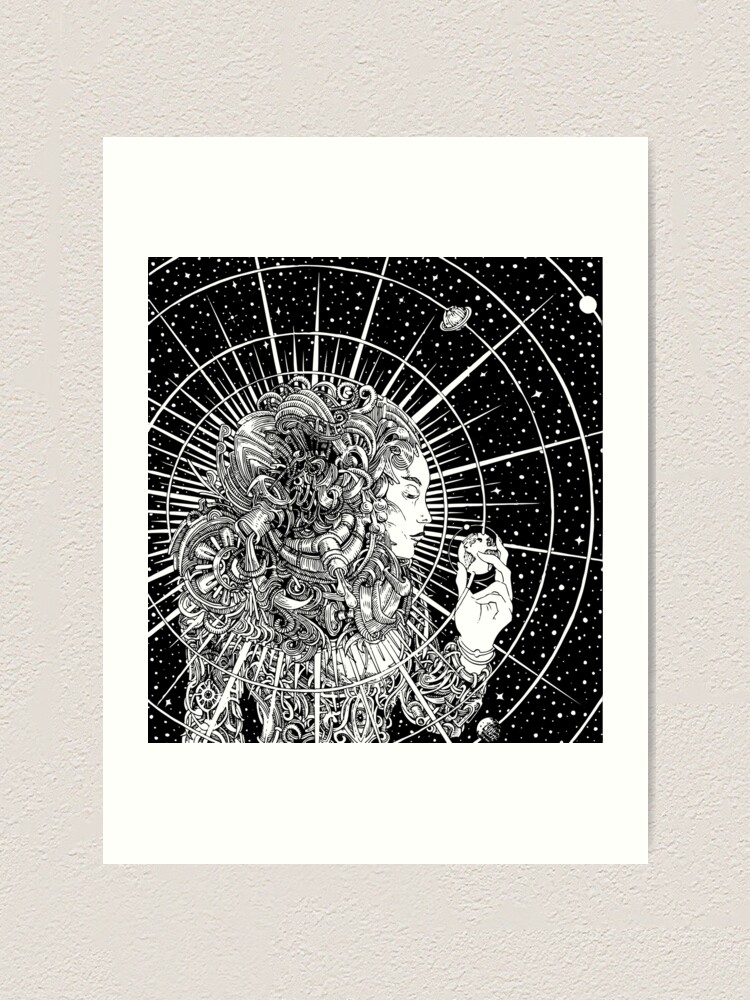The image is a black and white drawing centered on a vertically aligned rectangular piece of white cardstock, which is placed against a textured off-white wall. The drawing depicts a woman in the forefront holding what appears to be a small Earth or globe in her hand, which she grasps delicately with her first three fingers while looking at it intently. 

Her hair is wild and intriguing, composed of curls intertwined with mechanical elements such as gears, pouring objects, and possibly a wheel. She has a normal-looking face and hand, contrasting with her elaborate hair and outfit, which consists of chains, tools, and swirling metal patterns.

Behind her, a series of concentric circles radiate outward with rays emanating from them, resembling celestial or solar system elements. The background features white stars set against a black space, and in the upper-right part of the image, planets like Mars and Saturn—with its iconic rings—are visible.

The entire drawing sits on a white, square background within the vertically aligned rectangular cardstock, creating a striking juxtaposition of mechanical intricacy and celestial beauty.